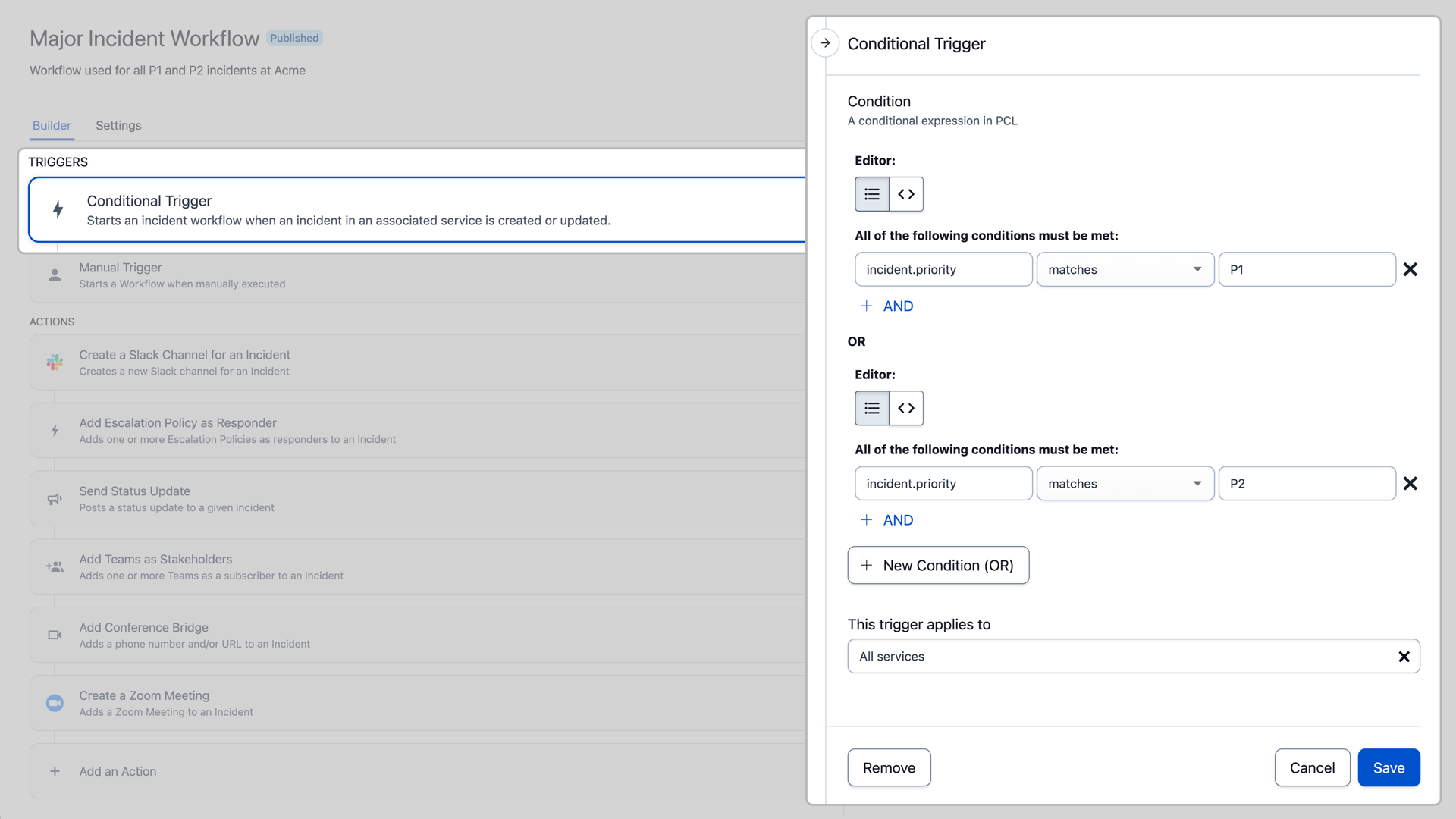Screenshot of the Major Incident Workflow Page

The image captures a screenshot of the major incident workflow page, predominantly characterized by a light gray background on the left side. A prominent white inlet box occupies the right half of the screenshot.

In the upper left-hand corner, the heading "Major Incident Workflow" is displayed, with the status "Published" noted beneath it in smaller text. The page specifies that this workflow is utilized for all P1 and P2 incidents at ACME. Below this header, the page indicates that the builder is currently selected, while the settings option is not selected.

The workflow section begins with "Triggers" and "Conditional Triggers," the latter highlighted by the white box on the right side of the image. The workflow further details the conditional trigger structure, starting with "Condition," which includes a conditional expression in PCL (Presumably “Process Control Language”). Following this, there is an "Editor" featuring various options, succeeded by an "Or" section with an additional editor and its own set of options. The white box concludes with options for adding a custom trigger, removing, canceling, or saving changes.

Toward the left side of the image, grayed out in the background, are additional options labeled for a manual trigger. These include actions to "Create a Slack Channel for an Incident," "Add Escalation Policy as Responder," "Send Status Update," "Add Teams as Stakeholders," "Add Conference Bridge," "Create a Zoom Meeting," and "Add Additional Action."